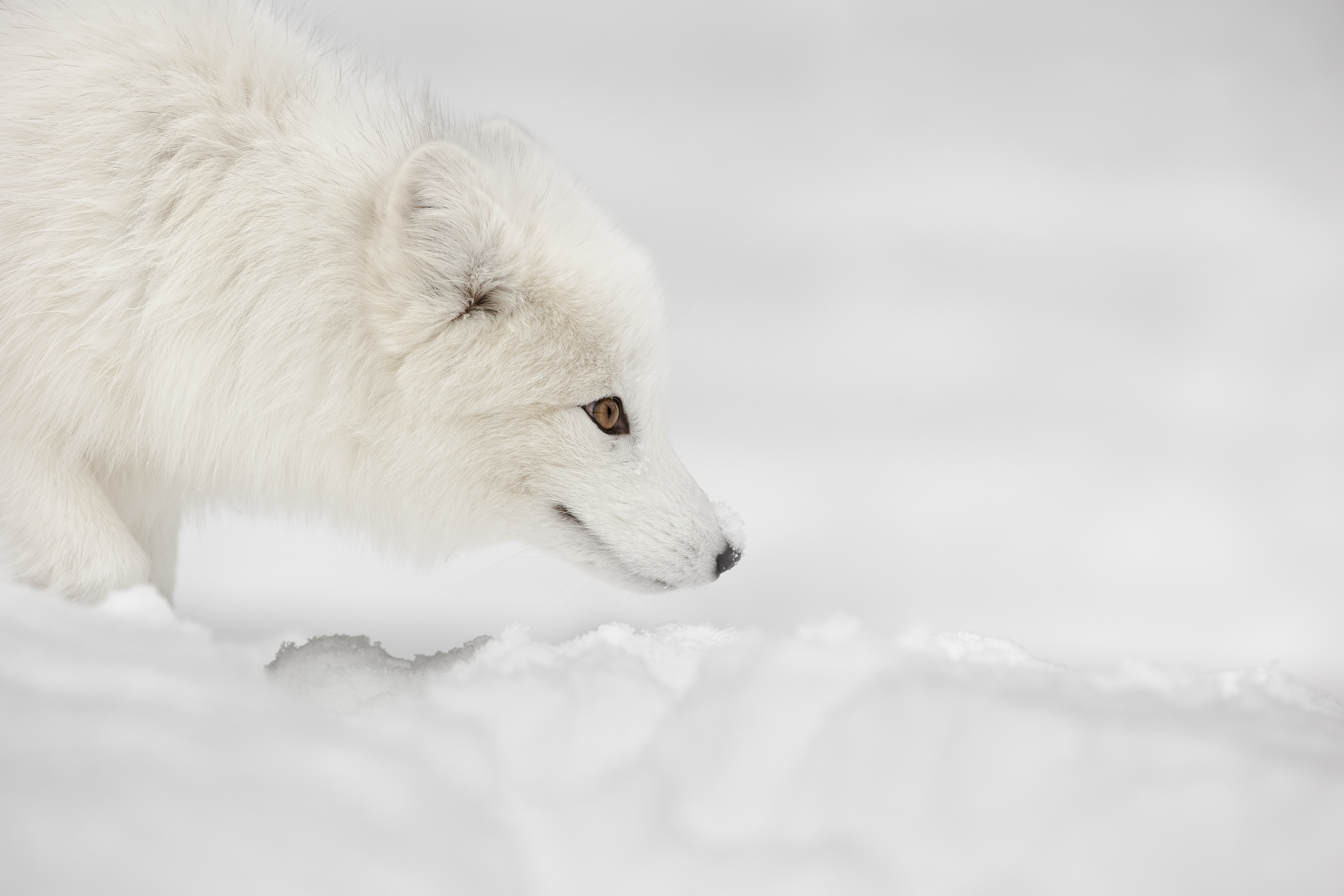This is a close-up photo of the front half of a white fox standing on snow in a snowy environment. The fox has thick, completely white fur with the exception of some dark fur inside one ear. Its hazel eyes are intensely focused forward, seemingly eyeing its prey. The fox's head is slightly bowed with its nose pointed toward the snow but its eyes looking straight ahead. The background is a blurred mix of grayish-white snow, creating a serene yet intense atmosphere. The fox's detailed features, such as its black and gray snout and the outline of its mouth, are clearly visible, adding to the meticulous depiction of the scene.